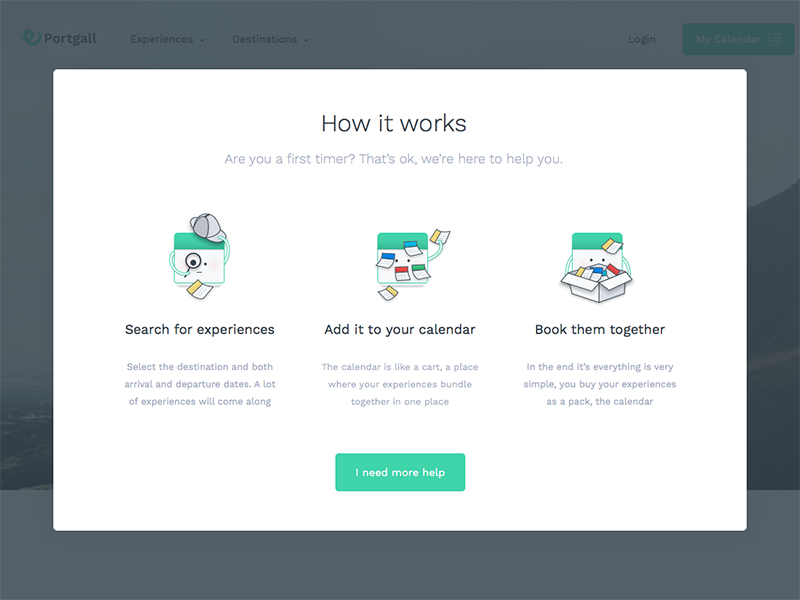The image shows a website with a darkened background, partially obscured by a large pop-up box. The visible parts of the website reveal it is from "PortGal," showcasing tabs for "Experiences," "Destinations," and "Login" on the right-hand side. A green box labeled "My" something is visible, along with a white bar at the bottom.

The pop-up box, taking up most of the screen, is titled "How it Works." It addresses first-time users with reassuring text: "Are you a first timer? That's okay, we're here to help you."

Below this text, the pop-up divides into three sections, each with detailed illustrations and descriptions:

1. The first section on the left, labeled "Search for Experiences," depicts a computer with a magnifying glass and a hat adorned with twigs for arms. A piece of paper appears in front of it. The accompanying text instructs users to search for experiences by selecting destinations and specifying both arrival and departure dates, promising an array of experiences in return.

2. The middle section, "Add it to Your Calendar," features an image of a computer with stick arms holding multicolored pieces of paper (blue, red, green, and gold). This section explains that the calendar acts as a cart where all chosen experiences are bundled together in one place.

3. The rightmost section, "Book Them Together," includes an image of a computer placing all the notes into a box. The text emphasizes the simplicity of purchasing experiences as a package and managing them in the calendar.

At the bottom of the pop-up, a green bar labeled "I Need More Help" offers additional assistance to users who require further guidance.